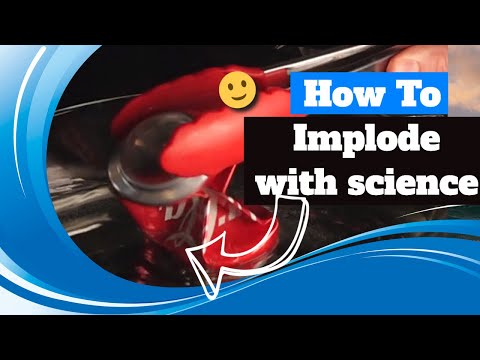In the center of the image, towards the top right, a person can be seen holding a pair of silver tongs. The ends of the tongs are gripping the bottom of a crumpled aluminum Coca-Cola can. The can is severely twisted and appears to be partially crushed. In the foreground to the right, bold white lettering spells out "How to Implode with Science," with a white arrow pointing directly at the Coca-Cola can. The can itself rests on a shiny stainless steel surface. A striking blue and white wave-like design sweeps diagonally from the top left to the bottom right of the image, adding a dynamic visual element. The image is framed with a black border at the top, and a very thin black border along the bottom.